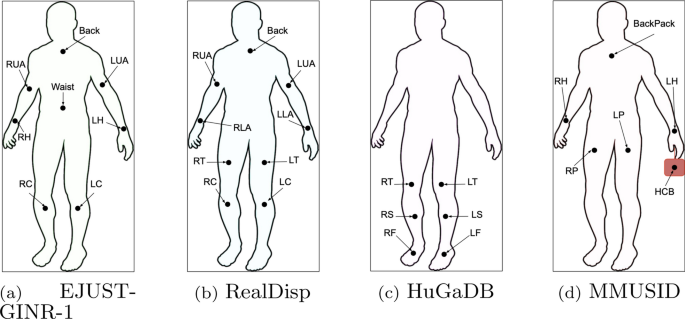This image is a detailed anatomical illustration taken from a textbook, depicting four sections of a human body outline, each labeled with specific annotations and titles beneath them. All sections are black-and-white line drawings set against a white background, showing standardized human body figures, likely male.

- **First Section**: Titled "A (EJUST-GINR-1)," it labels various body parts across the entire figure, including left and right knees, left and right hands, left and right upper arms (LUA, RUA), and the back. Additionally, it includes a label for the waist.

- **Second Section**: Titled "B (REAL-DISP)," this section is similar to the first but omits the waist and includes labels for the right and left thighs. It also notes right and left hands, upper arms, and the back (RH, LH, LUA, RUA).

- **Third Section**: Titled "C (HUGABD)," this section focuses on the lower part of the body, detailing areas from the thighs to the feet. It labels right and left thighs (RT, LT), knees, shins, and feet (RTR, RTL, RTF, LTF).

- **Fourth Section**: Titled "D (MMUSID)," it includes annotations for various body parts such as the right hand (RH), left hand (LH), left and right pelvis (LP, RP), and also shows a backpack. Additionally, there is a label near the hand marked HCB.

Each section has small black dots with arrows pointing to specific body parts, indicating focus areas that could be pressure points or other significant anatomical locations.